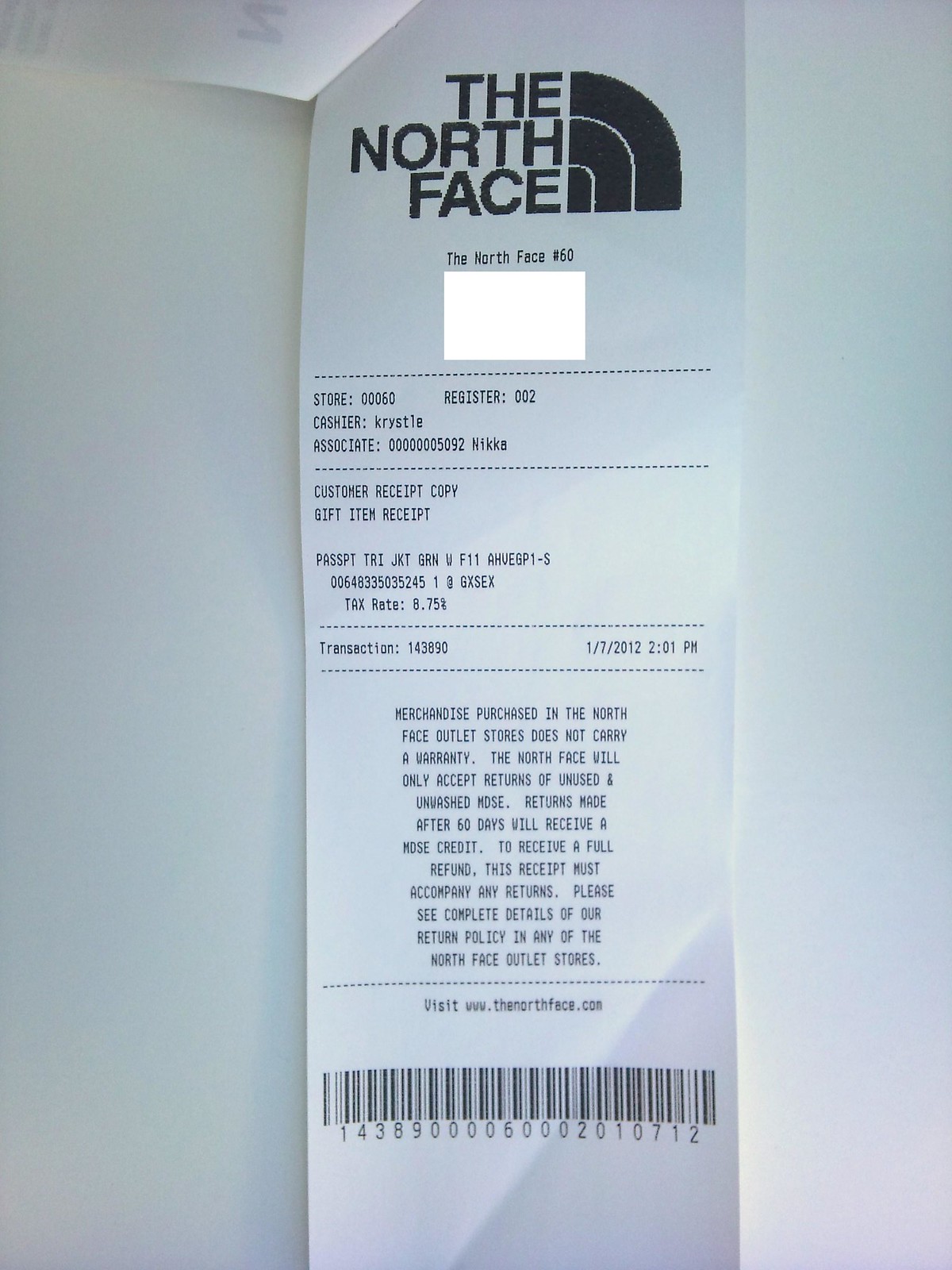This detailed indoor color photograph features a North Face store receipt displayed against a light gray or white background. The receipt indicates the transaction took place at store 0060, using register 002, with Crystal as the cashier. The date and time recorded are January 7, 2012, at 2:01 PM. Notably, this receipt is a customer gift item receipt, presumably for a jacket, although the price is not visible. At the top, "The North Face" is prominently displayed alongside the store’s logo, which consists of three partially arching thick lines.

The receipt features extensive information, including the transaction ID number 143890. At the bottom, it specifies the store’s merchandise policy: Items purchased at North Face outlet stores lack a warranty, and only unused and unwashed merchandise will be accepted for returns. Returns made after 60 days will be granted merchandise credit. To obtain a full refund, this receipt must accompany the return. More details on return policies can be found at any North Face outlet store or by visiting www.thenorthface.com. A long UPC barcode is also visible towards the bottom.